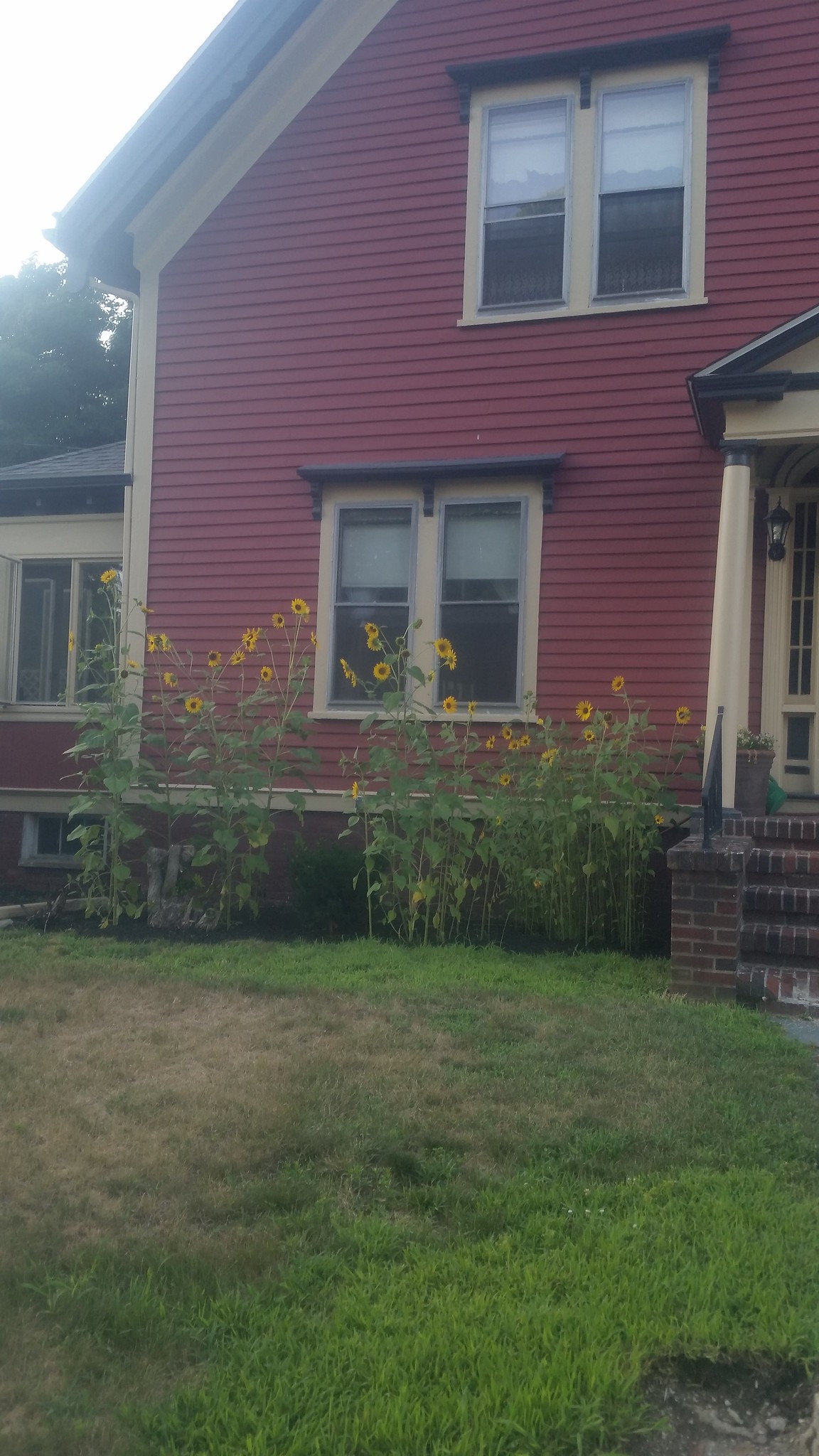This image captures a detailed view of an older two-story house with striking red siding reminiscent of brick, accented by white trim. The house's front facade features four windows with white frames, topped with black decorative elements. The roof, primarily dark with a distinguishing white outline, complements the structure's color scheme. To the right, a stone-brick staircase, bordered by white pillars, leads to the entrance sheltered by a small black roof. The forefront of the image showcases a well-maintained lawn with a line of tall sunflowers in full bloom just left of the entrance. A tree is visible behind the house, and sunlight from the back left casts a slight overexposure, adding a natural glow to the scene.